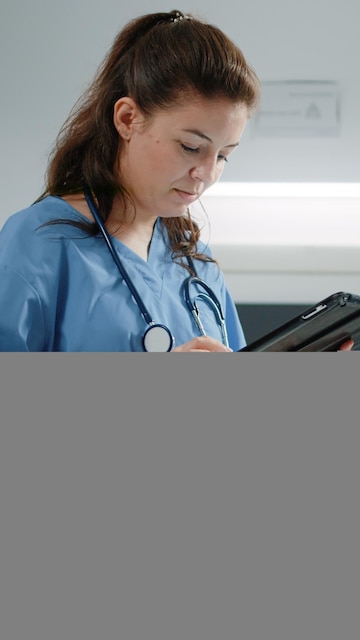The image features a middle-aged white woman in the medical field, likely a doctor or nurse, dressed in light blue scrubs. She is wearing a blue stethoscope around her neck, with the stethoscope's chest piece visible on our right side of the image. Her brown hair is styled in a half-up, half-down fashion, flowing down to a little past her shoulders. The nurse is looking intently at a black-covered iPad, which she holds subtly with her left hand. She has small stud earrings. The background is white and blurry, with a light source visible on the wall behind her, adding a sterile feel to the setting.